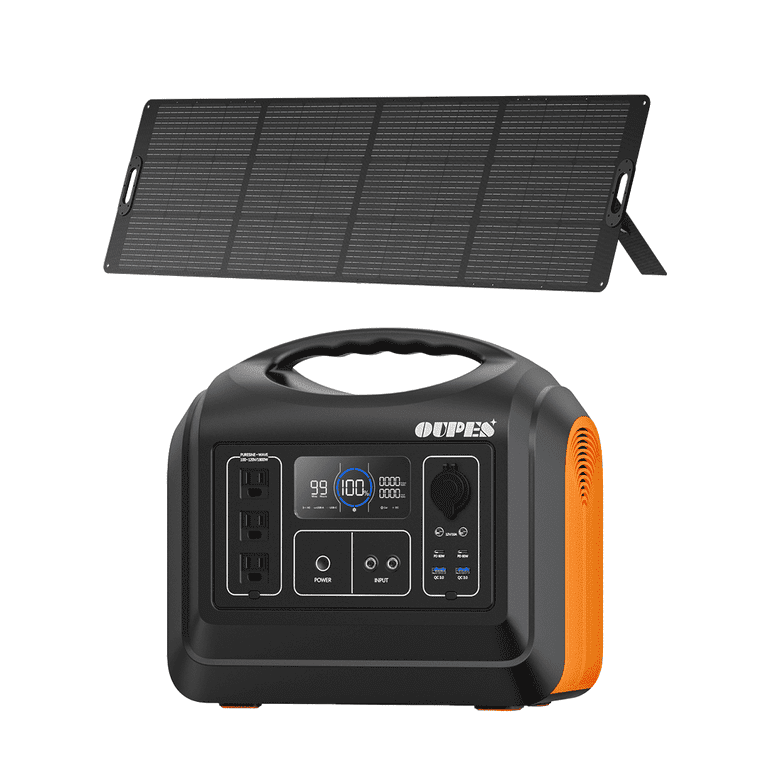The image is a detailed color photograph of a solar-powered generator used for product demonstration purposes, likely for online retail platforms such as Amazon. The image, in portrait orientation, features a portable black solar battery pack with a rounded handle on top and accents in orange and white. The black box, labeled "OUPES," showcases three standard three-pronged outlets on its left side, numerous USB and USB-C ports, along with a port for a classic car charger connection. Additionally, there's a digital meter on the top center that displays power status, indicating 100% charge capacity which decreases to 99%, and a rubber-capped input socket. 

Mounted above the generator is a large solar panel, tilted slightly towards the upper right, propped up by a visible support base. The panel is comprised of three rows of four solar cells each, extending across the top portion of the image from left to right. It features cutout holes for handles positioned in the middle on both the left and right sides. The background of the image is white, helping to focus attention on the floating equipment, and the photographic style captures the realistic and functional aspects of the product.